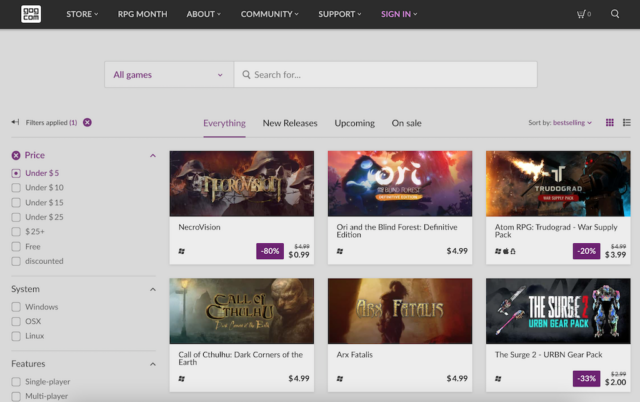Screenshot of a Video Game Website:

The screenshot features a website for video games with a clean and organized interface. At the top of the page, there is a black navigation bar which includes menu options such as "Store," "RPG," "A Month," "About," "Community," and "Support", each accompanied by a downward arrow indicating a dropdown menu for further selections. To the far right, highlighted in purple, is the "Sign In" button.

Beneath this navigation bar is a section depicting a shopping cart icon, followed by a prominently displayed "All Games" heading and a search bar for easy game discovery. The background of these elements is a neutral gray, which complements the purple text accents and makes them stand out.

On the main section of the page, six different video games are showcased, each with their respective prices listed next to them. Adjacent to the game listings is a vertical navigation menu that allows users to filter games based on price categories: "Under $5," "Under $10," "Under $15," "Under $25," and "Above $25." 

Further down, the filters continue with system compatibility options including "Windows," "OS X," and "Linux." Another filter section follows, categorizing games based on features such as "Single Player" and "Multiplayer."

The games listed are:
1. NecroVision
2. Ori and the Blind Forest
3. Atom RPG
4. Chateau
5. The Surge – Urban Gear Pack

Overall, the layout is user-friendly, with clear categories and filters to enhance the browsing experience for video game enthusiasts.